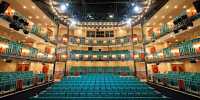The photograph depicts the interior of a brightly lit, multi-level theater, though the small size and distance make details hard to discern. Predominantly featuring hues of turquoise, gold, red, and some black, the image shows rows of teal seats extending across the floor, likely for audience members. The theater appears to have three tiers on either side, which might be balconies or private boxes adorned with green, red, and yellow coloring. Bright white lights are scattered throughout, illuminating the space prominently. The photo seems to be taken from the stage, looking outward, capturing the grandeur and vivid color scheme of the interior, but the specifics remain somewhat fuzzy due to the image's diminutive size and resolution.